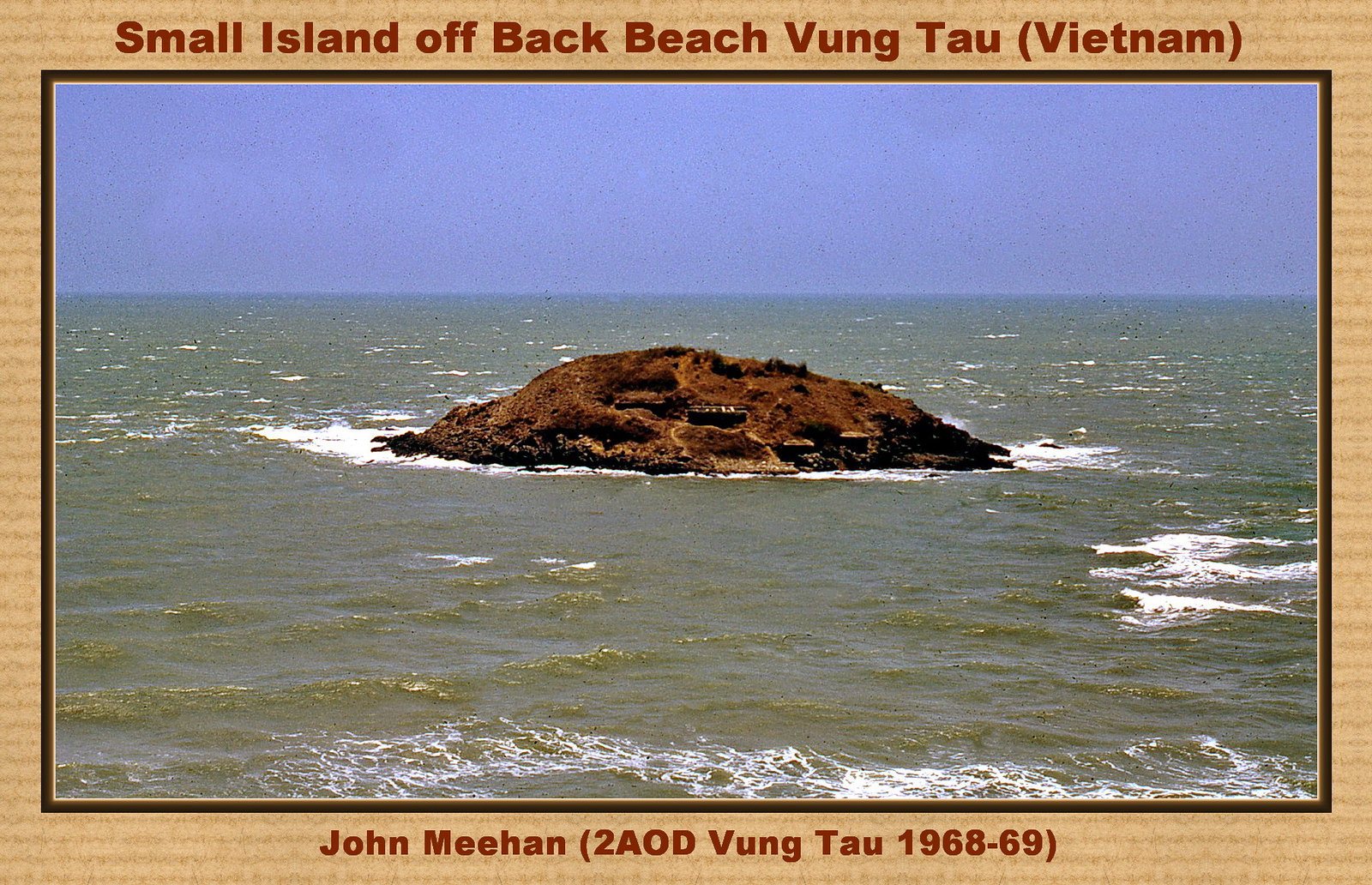This photo, resembling a vintage postcard with a tan frame, depicts a small, dome-shaped island centered within a green ocean. The island, primarily composed of brown rock and stone, features some sparse grassy growth. Several structures, including one larger flat-roofed building with a black opening and two smaller huts, are visible on the island. Gentle waves with white foam lap against the rocky shoreline. Above the serene scene, the sky transitions from a light blue to a berry tone. The caption at the top of the postcard reads "Small Island off Back Beach, Vung Tau (Vietnam)," while the bottom inscription states, "John Meehan (2AOD, Vung Tau, 1968-1969)."